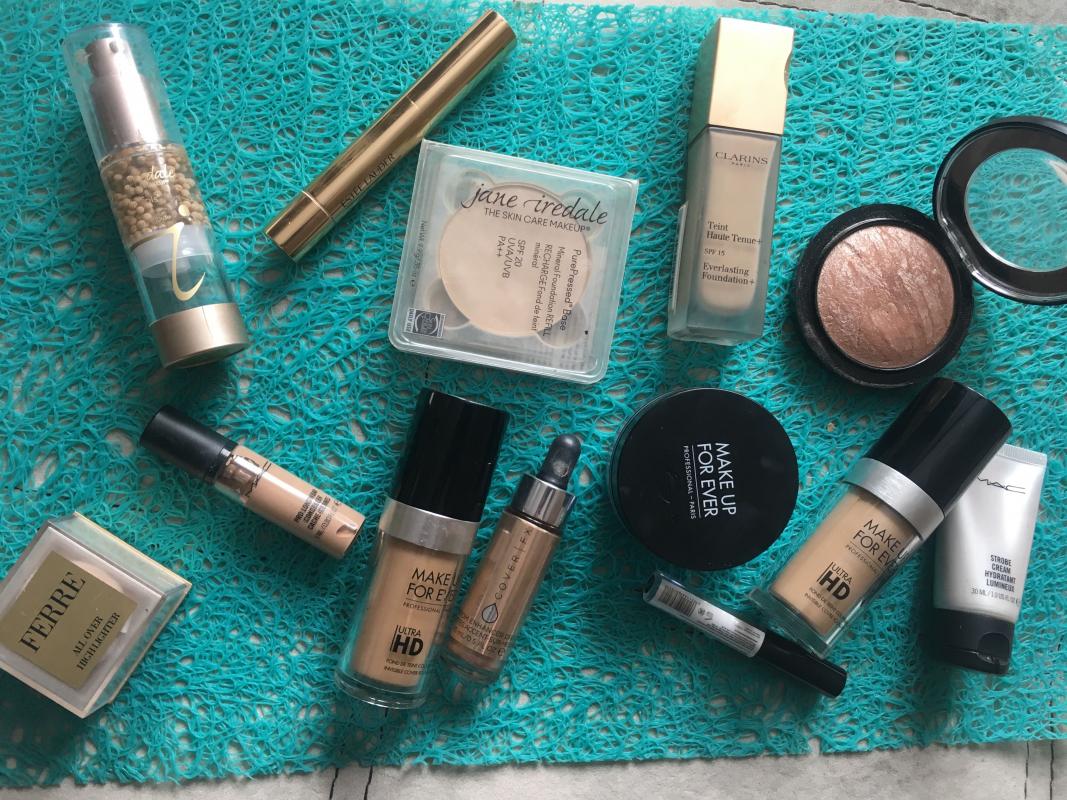The image showcases an assortment of makeup products elegantly arranged on a white counter covered with a delicate, blue, lacy, and semi-transparent fabric that reveals parts of the table beneath. The detailed layout includes:

- **Top Left Corner**: A plastic tube slightly angled to the left with a silver nozzle, clear cap, and small brown pellets inside. A green clear section adorned with a silver 'J' and a silver bottom completes the tube.

- **Above to the Right**: A silver, or possibly gold, eyeliner with its end pointing up to the right diagonally.

- **Below the Eyeliner**: A clear square box containing brown foundation.

- **To the Right of the Foundation Box**: A rectangular tube with a gold top, filled with brownish foundation-like content.

- **To the Right of the Rectangular Tube**: An open mirror, with its reflective surface propped up to the right, encased in a black frame.

- **Below the Mirror**: A broad makeup tube with a black cap, a silver middle section, and a visible brown substance inside.

- **To the Right of the Broad Tube**: A silver tube with a makeup product, featuring a black-capped end pointing downward.

- **Below the Broad Tube**: A slender tube with a black cap positioned downward to the right, its label visible and tilting upward to the left.

- **Above the Slender Tube**: A small, round, black makeup tub.

- **Two Larger Tubes Nearby**: Both have black tops and silver middle sections; one is capped, while the other is not.

- **Adjacent to These Tubes**: Another square makeup container with a gold top labeled "F-E-R-R-E" in black lettering.

Each product, with its distinct packaging and color scheme, adds to the rich texture and variety of the makeup collection displayed.